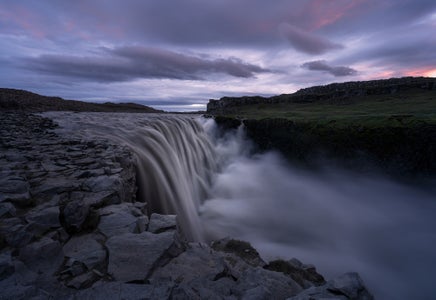The image portrays a captivating nature scene, potentially a painting due to its intricate details and vivid colors. Dominating the center is a powerful waterfall cascading down from a rocky cliff, with robust streams of water forcefully hitting the rocks below, creating an impressive mist and turbulence. The waterfall is framed by imposing rock formations on both sides, adding depth and a sense of grandeur.

The sky above suggests a dramatic sunset with a palette of purplish-blue and pink hues. The clouds are thick and heavy, mostly clustered together, although a few drift independently, contributing to the overall intensity of the sky.

To the right of the waterfall, the terrain is rugged with scattered rocks, while the left side reveals a lush, green island or cliffside, adding a touch of verdant vitality to the composition. The scene is dark and atmospheric, with dark blues, blacks, and grays giving it a somewhat somber, twilight feel. The mist and steam rising from the waterfall enhance the mystical and serene ambiance, capturing a moment of natural splendor frozen beautifully in time.